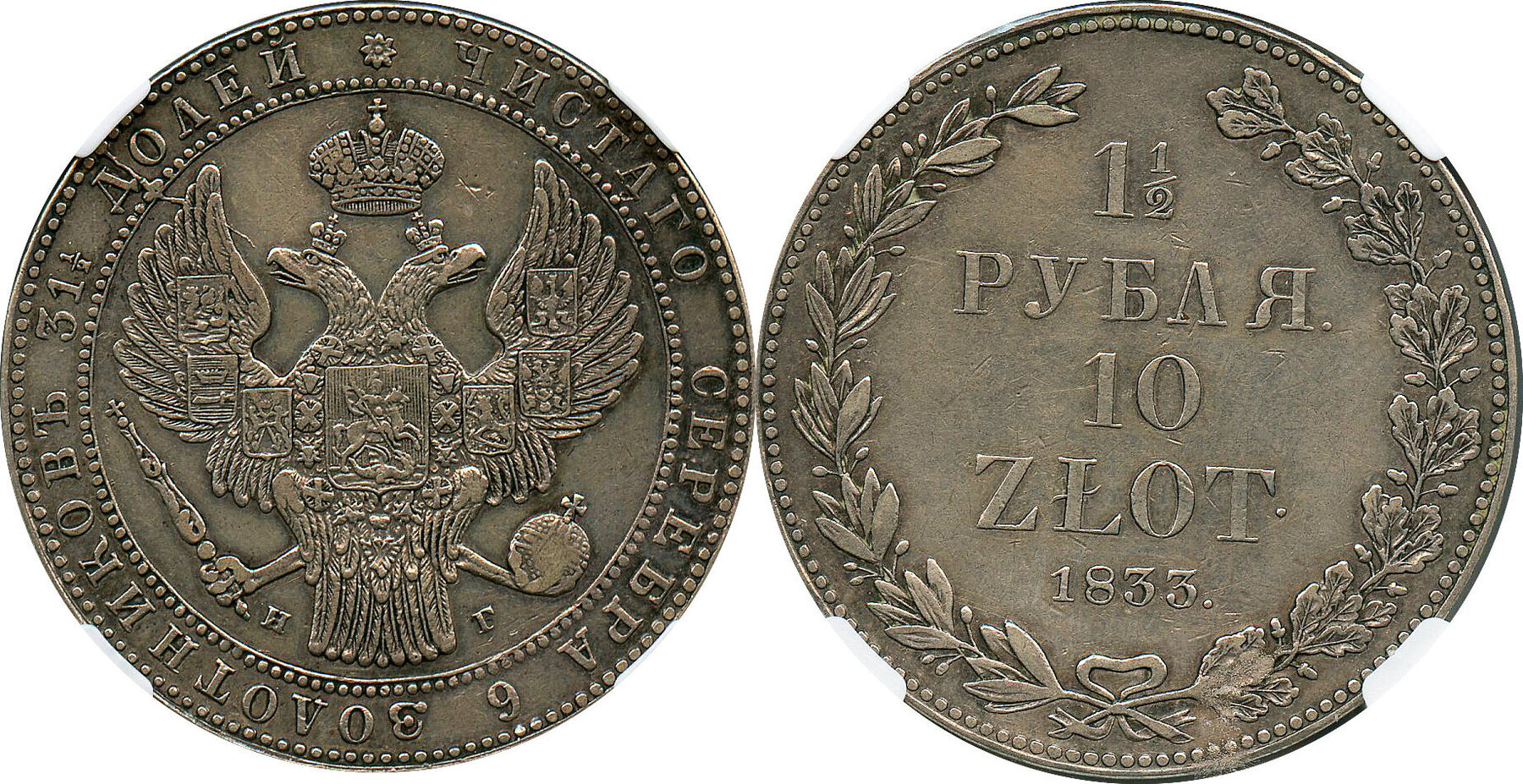This image depicts the front and back of an antique coin set against a completely white background. The coin, possibly Russian, showcases intricate details and text in a foreign language. The front side features a double-headed eagle, each head adorned with a small crown, and a larger crown above them. The eagle's right talon clutches a round orb with a cross, while the left talon grips a scepter topped with a cross. Encircling this detailed imagery is an inscription in an unfamiliar script, bordered by a ring of small beads, with noticeable chipping on the edge. The reverse side prominently displays the numerals "one and a half" followed by another foreign word, then "ten", "zlot", and the date "1833", all framed by an ornate laurel wreath decorated with numerous leaves and buds. The coin is silver in color with a textured edge, exuding a sense of age and historical significance.